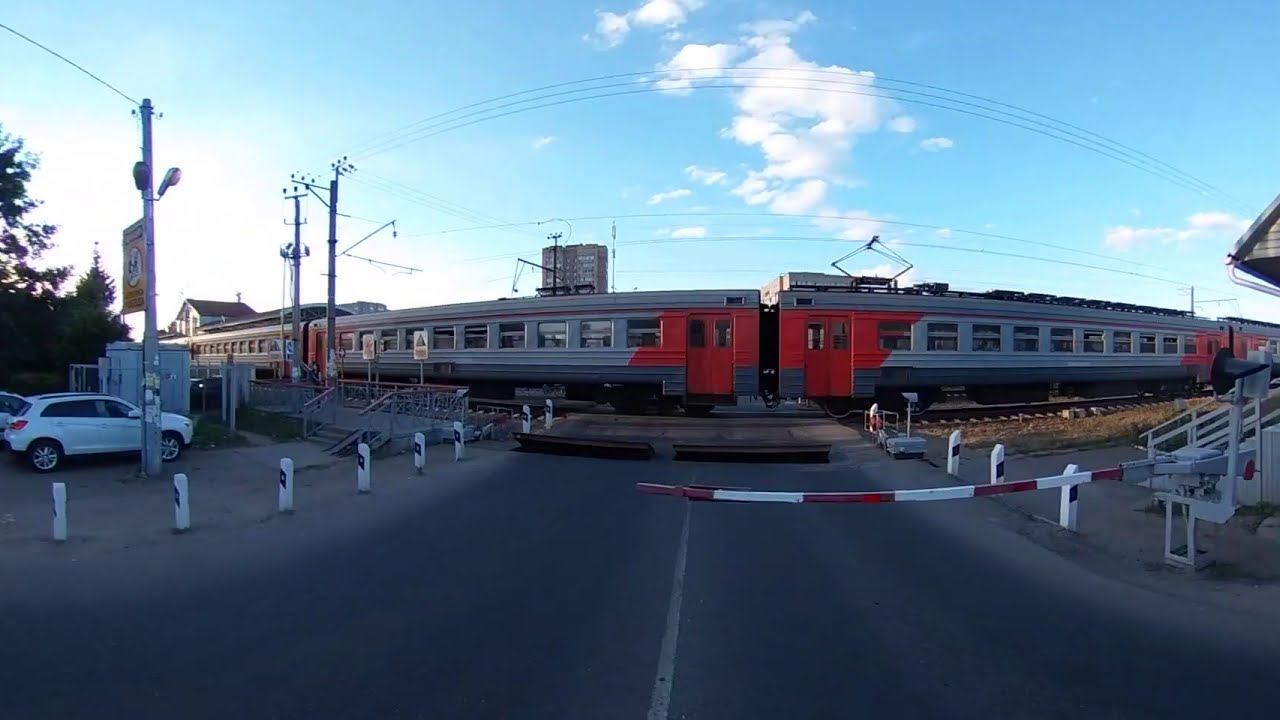The image captures a detailed outdoor scene of a gray train with orange and red accents, prominently situated in the background. The train, which appears to have a lighter gray top and darker gray bottom, travels along railroad tracks under a light blue sky scattered with a few white, wispy clouds. A red and white striped crossing bar is lowered, blocking a road that cuts through the foreground, divided by a white stripe down the middle. Flanking both sides of the railroad crossing are various white barriers and small posts. On the left side of the image, a white SUV is parked near parking spaces delineated by white lines, some of which are coned off with red and white ropes indicating no parking zones. Also on the left side are several power poles and power lines running horizontally above the train.